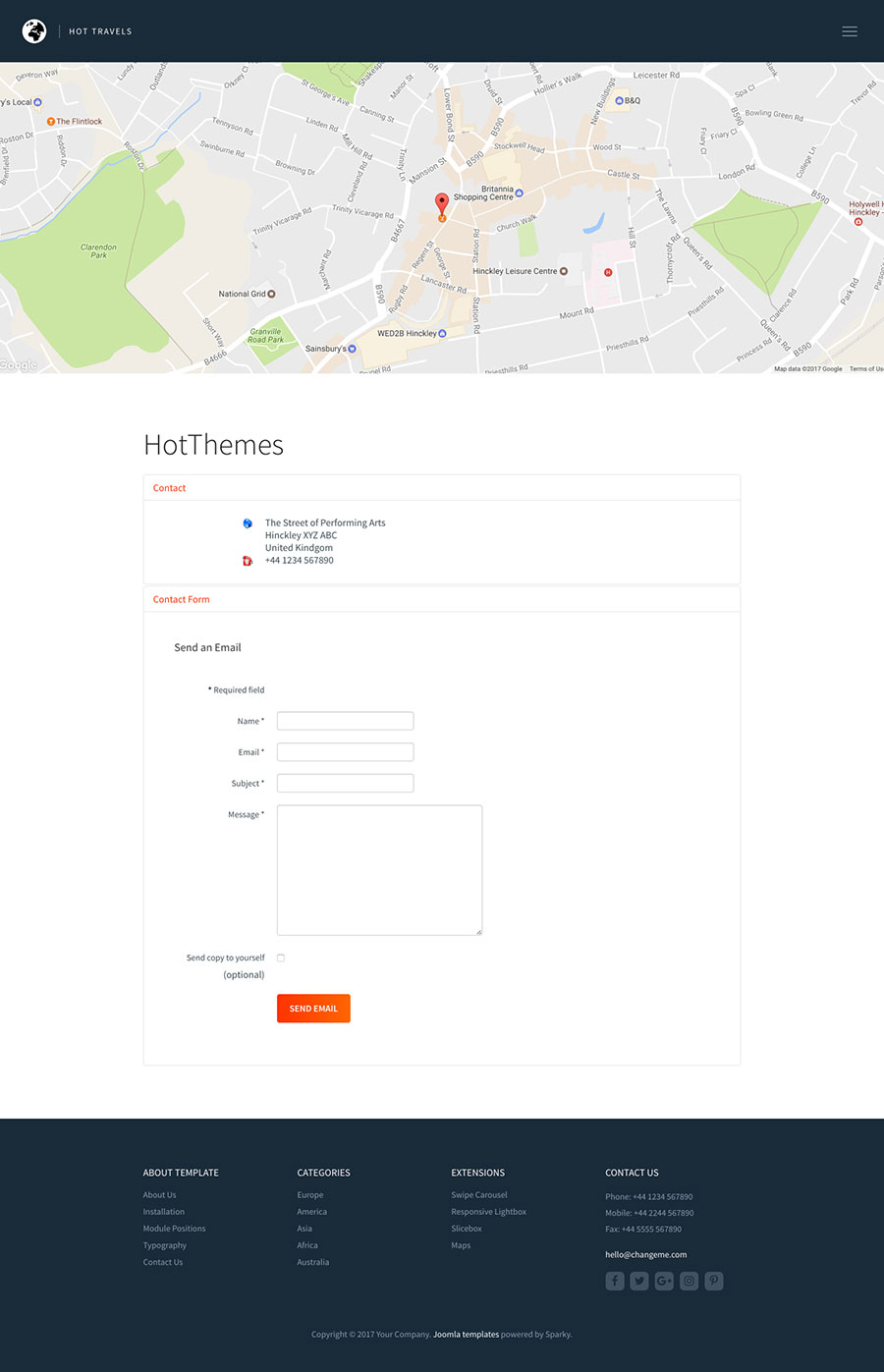The detailed caption for the image is as follows:

"This is a full-color screenshot of a website, which could be displayed on a laptop screen, computer monitor, or mobile phone. At the very top, there is a solid horizontal rectangular banner filled with black. On the right side of this banner, there is a spherical icon depicting countries in black. To the right of this icon, the text 'Hut Travels' is written in white letters.

Beneath the banner, there is a section featuring a map of the Britannia Shopping Center. This map shows light green patches representing areas of greenery, along with marked roads. A red teardrop marker indicates a specific location on the map. Directly below the map, there is a heading that reads 'Hot Themes.'

Further down, there is a box bordered in light gray. Within this box, the text 'Contact' is displayed in bold orange letters. Below this, the address reads, 'The Street of Performing Arts, Hinckley, ABC, XYZ, ABC, United Kingdom,' followed by a phone number. Below the address, in orange letters, it says 'Contact Form, Send an Email.' 

The form fields labeled 'Name,' 'Email,' 'Subject,' and 'Message' are laid out clearly for users to fill out. At the bottom of this section, a solid orange horizontal box features the text 'Send Email' in white letters, indicating where users can click to send their message."